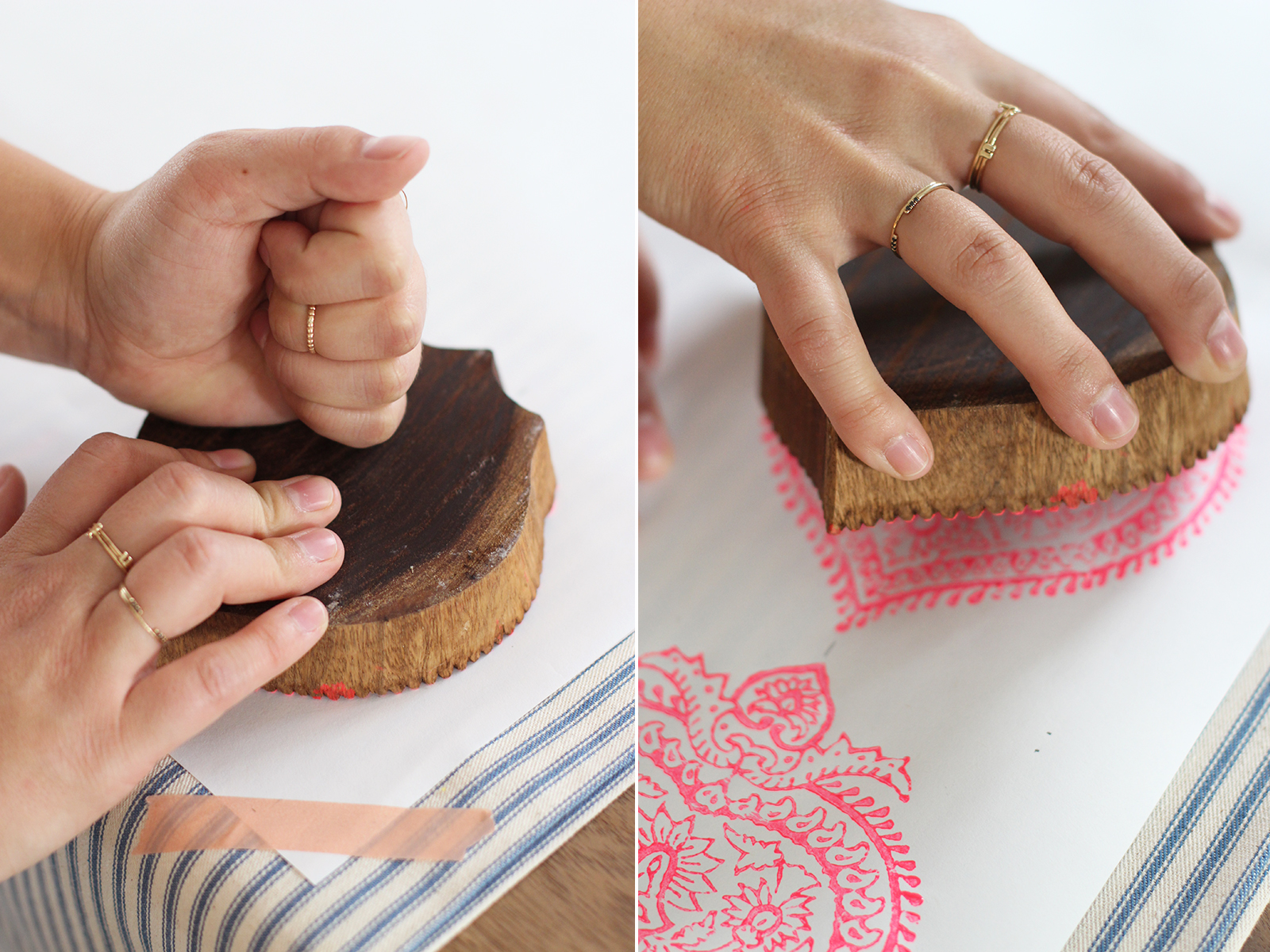This image, arranged in landscape layout, consists of two side-by-side vertical (portrait orientation) photographs separated by a thin white line, comprising a detailed scene of a stamp-block crafting process. In the left photograph, a Caucasian person's hands, adorned with gold rings, are engaged in the act of stamping a design onto white paper using a circular wooden stamp. The white paper is securely fixed with pink tape on a blue and white striped tablecloth, revealing a corner of the wood table underneath. The person’s right hand is balled into a fist pressing down on the top of the wood slice, while the fingertips of the other hand stabilize it from below.

The right photograph shows the same hand slightly lifting the wooden stamp, uncovering a vibrant pink heart imprint that the stamp has left on the paper. In the lower left-hand corner of this photograph, another identical pink heart stamp is visible. The overall setup, including the blue and white striped tablecloth and the pink accent details, suggests an engaging and creative stamp-making activity, captured in photographic realism style.